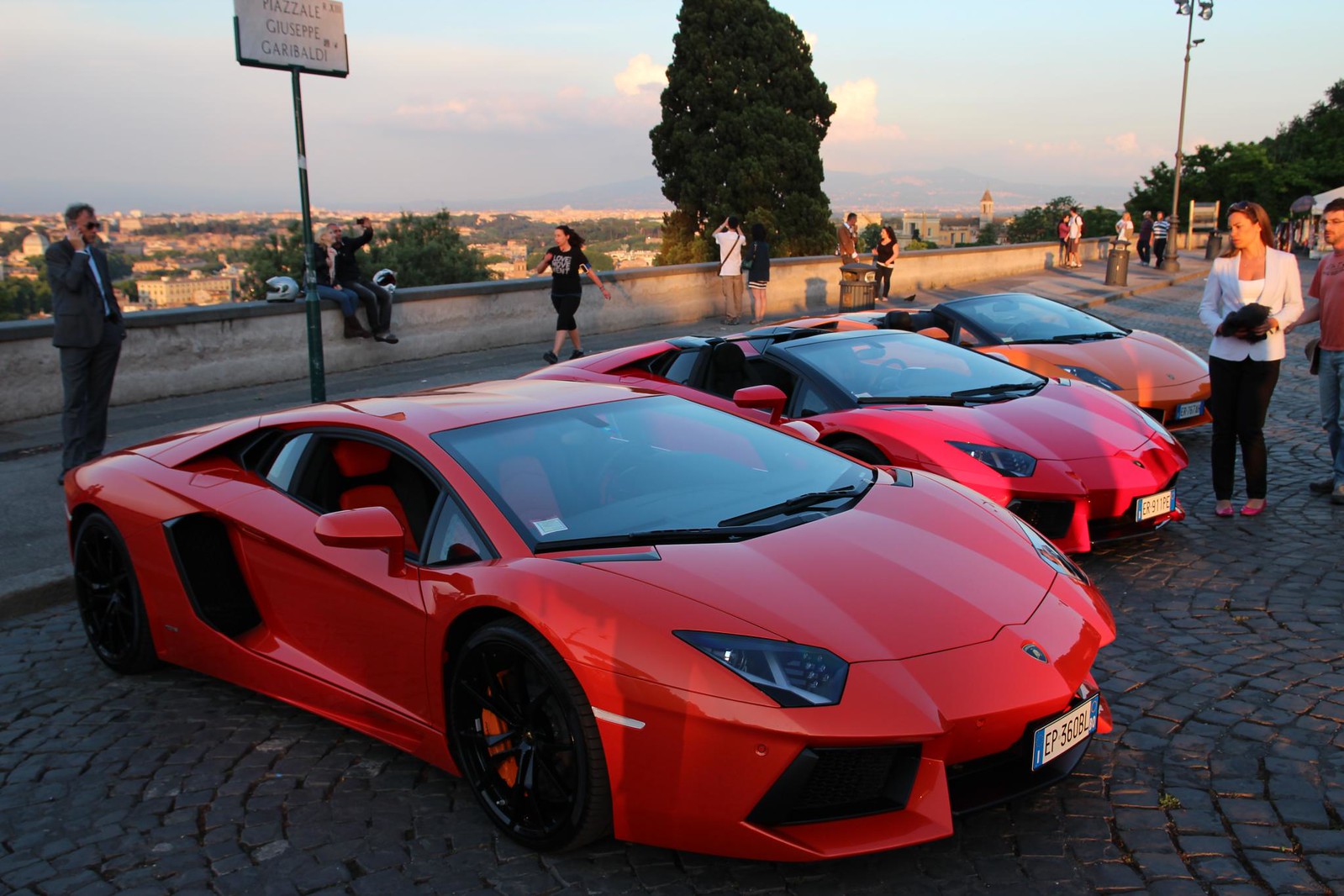In this image, you see three high-end, luxury sports cars that are likely Ferraris or Lamborghinis, aligned in succession on a decorative cobblestone street. The first two cars, closest to the photographer, are a vibrant red, while the third one, further in the background, is an eye-catching orange. The first car, with its top on, is situated closest to the left, while the second car, with its roof off, is positioned slightly behind and to the right of the first. The third car, also a convertible like the second, is a bit farther back and to the right.

The walkway behind the cars has multiple people strolling, with some taking particular interest in the vehicles. Specifically, a couple on the right-hand side is focused on the middle car; the woman, dressed in a white blazer, white tank top, black pants, and possibly red shoes, holds something black in her hand. Beside her, a man in a red T-shirt and blue jeans stands. On the far left of the image, a man dressed in a business suit and wearing glasses appears to be talking on his cell phone.

The backdrop features a scenic overlook of a city, accentuating a European vibe with visible elements such as a tree, a light post, and a barely readable sign behind the first car. The overall setting suggests a picturesque, possibly urban, locale that could be hosting a car show or similar event.